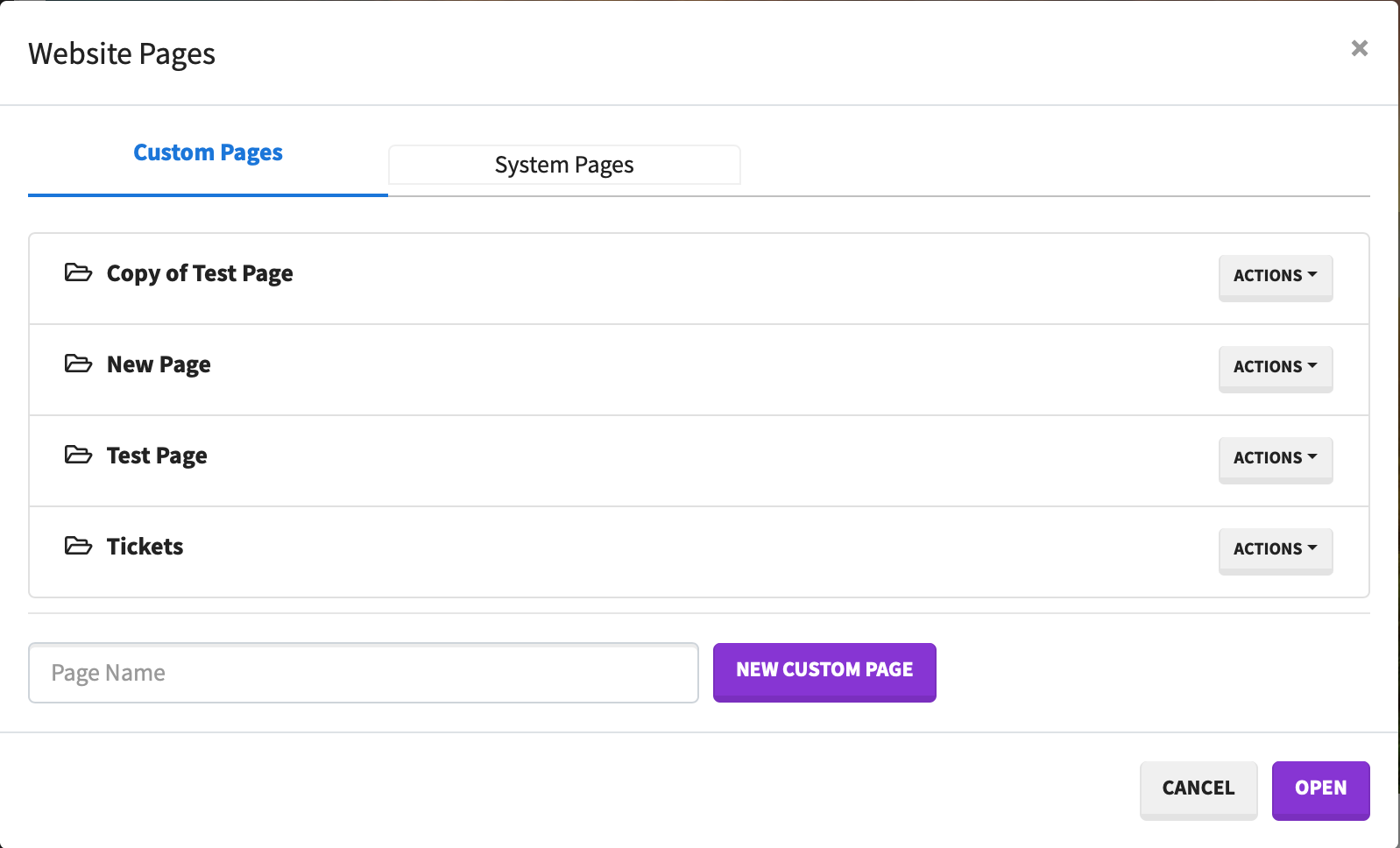This image depicts a webpage interface focused on managing website pages. In the upper left-hand corner, the text "Website Pages" is prominently displayed. The interface is bounded by a thin black border that spans the top and right sides but is absent on the bottom and left sides. Directly across from "Website Pages" in the upper right, there is a slightly grayed-out 'X' icon.

Below "Website Pages," a thin horizontal line separates the header from the main content. The section immediately below this line is divided into two tabs. The tab labeled "Custom Pages" is highlighted in blue, signifying its active status, with an underline beneath it. Adjacent to this, the "System Pages" tab appears as a white button.

The main content area is structured with four rows, each beginning with a folder icon. These rows represent different pages and include action buttons with drop-down arrows on the right-hand side. The rows are labeled sequentially as: "Copy of Test Page," "New Test Page," "Test Page," and "Tickets."

Beneath these rows is a smaller section with a sparse white area, accentuated by a single line. Following this is a rectangular area displaying the text "Page Name." To the right of this section, another smaller rectangular button labeled "New Custom Page" is visible.

At the bottom right corner of the interface, there are two additional buttons— "Cancel" and "Open." These buttons likely serve as actions related to the selection or creation of website pages.